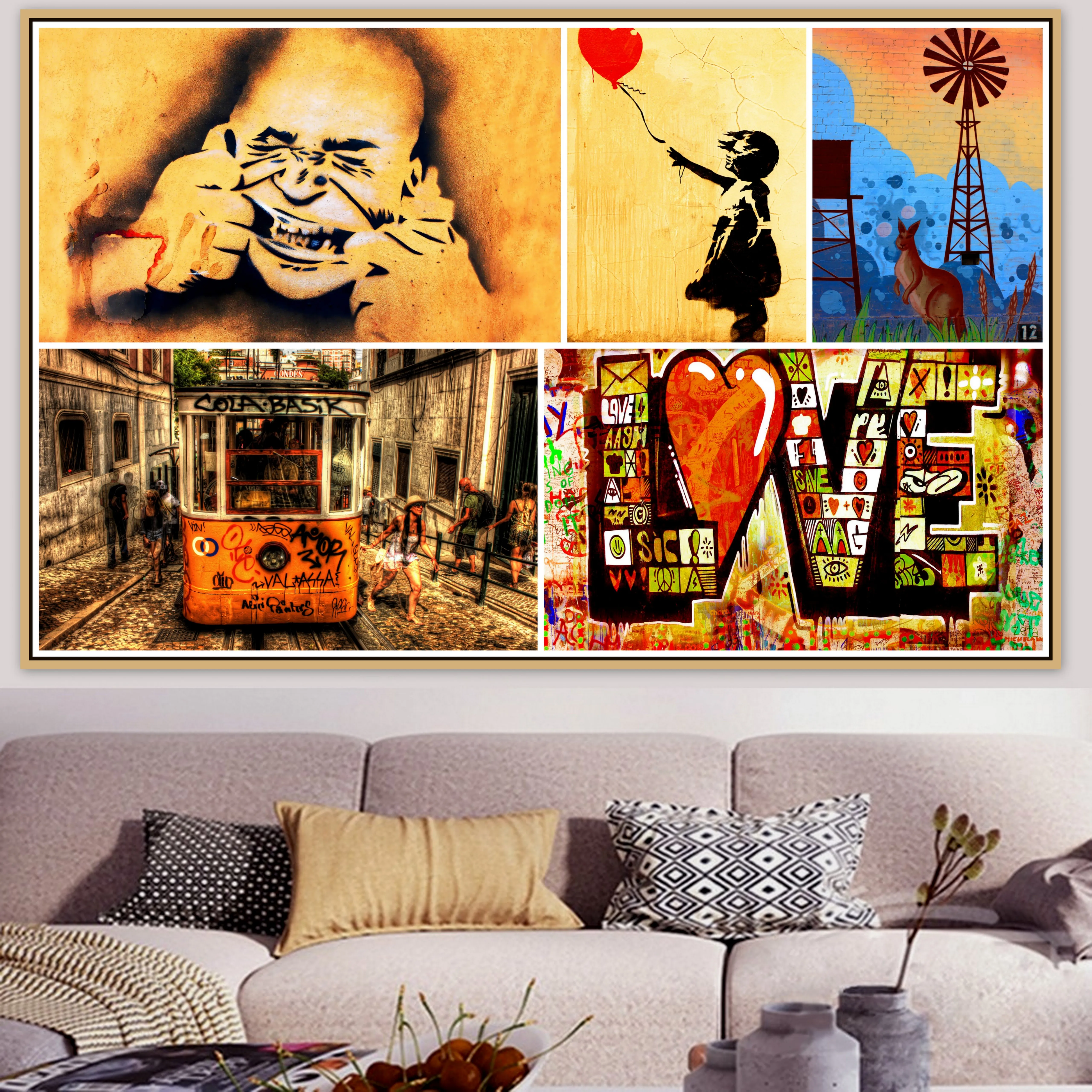In a cozy indoor setting, a light gray, overstuffed couch adorned with various pillows takes center stage. Among the pillows, one features black and white polka dots, another is a vibrant yellow, and a third black and white pillow showcases a diamond pattern. Draped casually over the couch is a beige throw blanket. In front of the couch, three gray vases are displayed, with one holding flowers and another accompanied by a white bowl filled with cherries, complete with green stems. Beside these vases, there is also a stack of books or magazines.

Above the couch hangs a captivating painting divided into five distinct sections. The upper left quadrant portrays a man stretching his cheeks to reveal his teeth, rendered in a yellowish-gold hue. Directly below is a street scene featuring a graffiti-covered trolley car with people nearby. The upper right section is split, presenting a black and white drawing of a young girl holding a red balloon against a yellow background, and next to it, a vivid outdoor scene with kangaroos and a windmill under a blue sky. The bottom right quadrant artistically spells out the word "LOVE," with the "O" depicted as a red heart. Each section of the painting adds a unique, dynamic element to the overall ambiance.